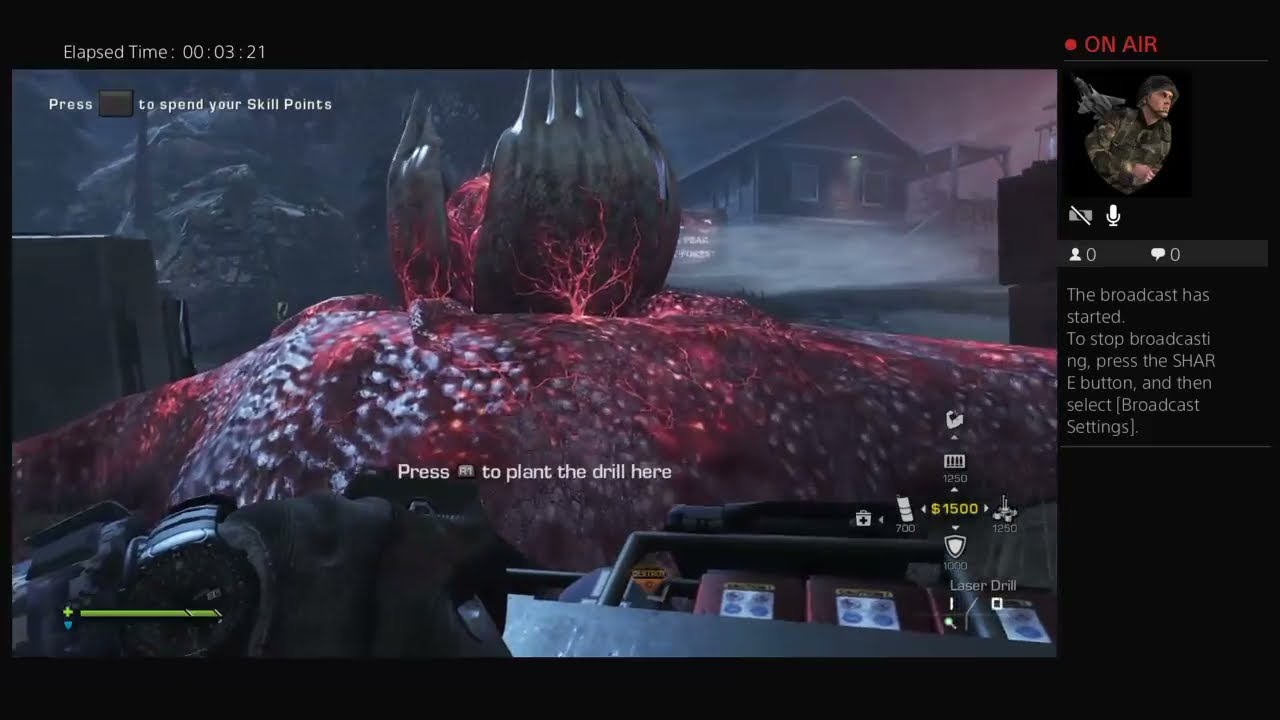This screenshot from a video game reveals a first-person shooter perspective, where the player, seen wearing black gloves and a watch, is equipped with a rifle. Dominating the dark gray sky background are two fog-covered structures resembling sheds or houses. At the center is a surreal, purplish, and red glowing mound, reminiscent of a volcanic formation, with tendrils extending from a large alien egg-like structure that is opening to reveal a pulsating red and purple core. Overlaying the scene is an assortment of in-game HUD elements: white text prompts the player to "press F1 to plant the drill here" and to "press a key to spend your skill points," while the elapsed time of 00:03:21 is displayed. In the upper right corner, red text indicates "On Air," with a soldier icon and a microphone below, accompanied by instructions, "The broadcast has started. To stop broadcasting, press the share button and select broadcast settings." Additionally, a health status bar with a green cross is situated in the bottom left corner of the screen.